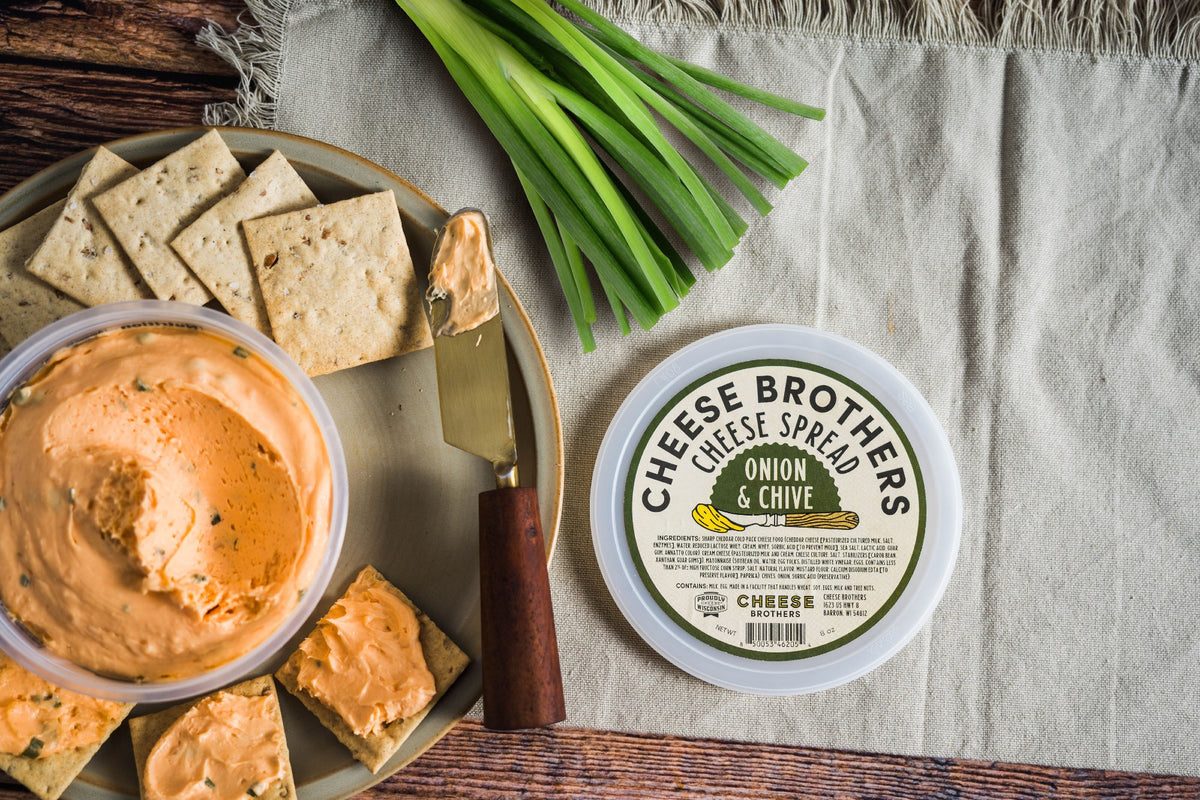The scene depicts a rich brown medium-tone wooden table as the backdrop. On the right side, there is a light gray textile placemat with frayed edges. Atop the placemat, there is a small, white circular container with a label that reads "Cheese Brothers Cheese Spread, Onion and Chive," featuring an illustration of a cheese knife. In the upper left corner of the placemat, a cluster of vibrant green chives rests, adding a pop of color. On the left side of the scene, a slightly darker gray plate with a gold rim holds square white crackers, several of which are topped with the yellowish-orange cheese spread. Positioned on the plate is a cheese knife, coated with the spread and evidently used, as indicated by a noticeable gouge in the container of cheese spread. The entire setup presents a visually appetizing tableau, combining rustic elements with a touch of elegance.